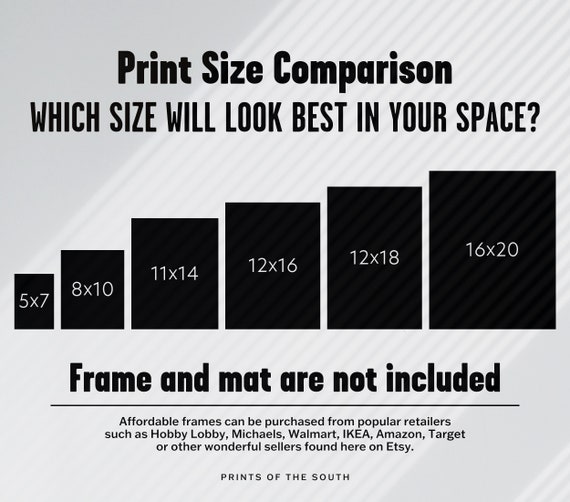The image is a simple, square-shaped black-and-white chart with no border, set against a gray background featuring white diagonal lines stretching from the lower left to the upper right corner. At the top, bold black text reads "Print Size Comparison" followed by the question "Which size will look best in your space?". The center of the image includes a bar graph with six black bars of increasing size from left to right, labeled with white text showing dimensions: 5x7, 8x10, 11x14, 12x16, 12x18, and 16x20. Below the bar graph, it states in concise text, "Frame and mat are not included." Further down, it mentions the availability of affordable frames from retailers like Hobby Lobby, Michaels, Walmart, Ikea, Amazon, Target, or other sellers on Etsy. Across the bottom of the image, the text "Prints of the South" is elegantly scripted.